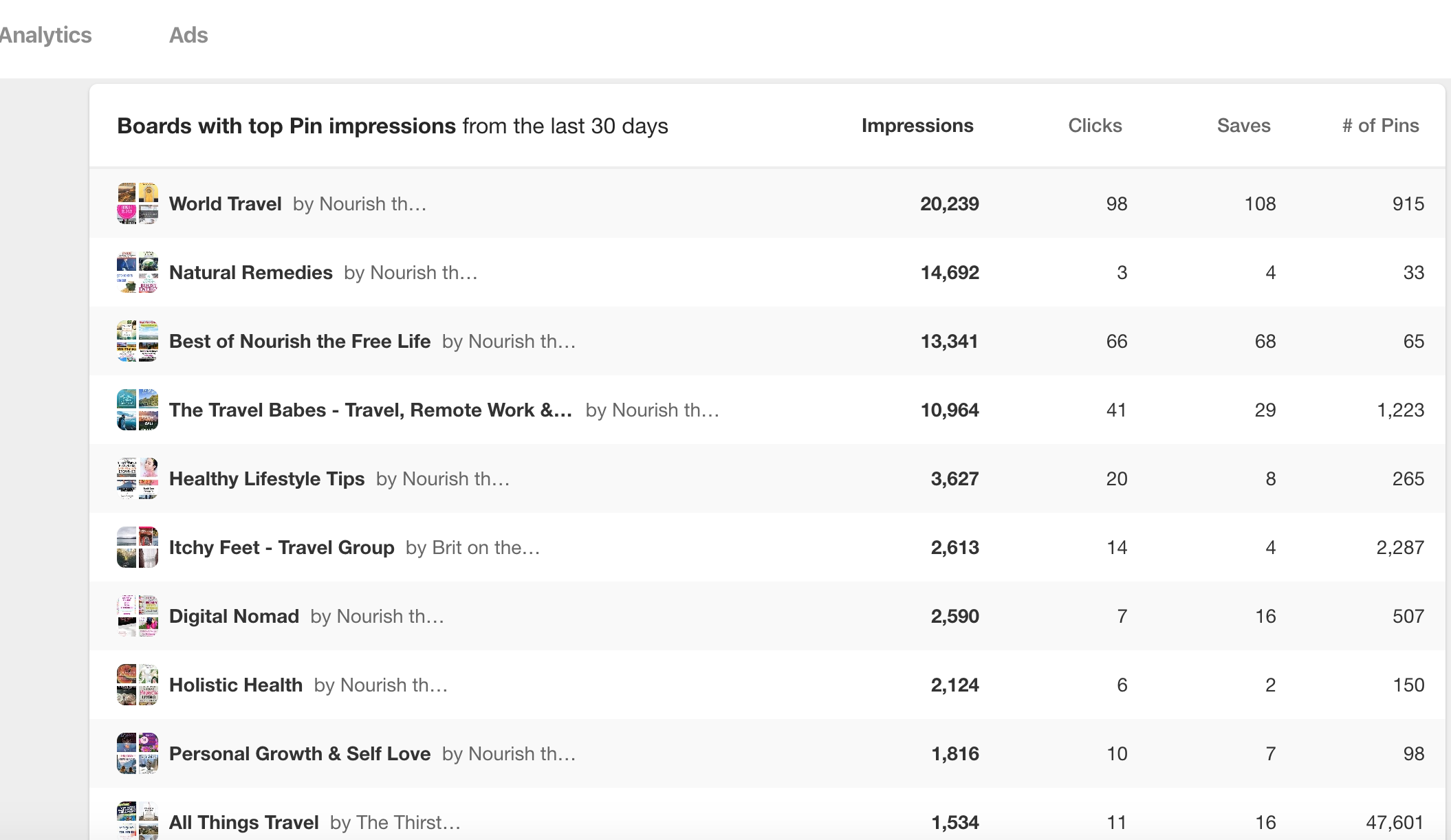**Detailed Web Page Screenshot Analysis: Analytics and Ads Overview**

The image showcases a web page predominantly characterized by a large white background. Positioned at the top left corner, the title "Analytics and Ads" is displayed prominently in black lettering. Below the title, in bold black text, is the heading "Boards with Top 10 Impressions from the Last 30 Days," highlighting the content's focus.

On the top right corner of the page, there are four key performance indicators listed: "Impressions," "Clicks," "Saves," and "Number of Pins."

The detailed breakdown of the top 10 boards with their respective statistics is as follows:

1. **World Travel by Nourish:**
   - **Impressions:** 2,239
   - **Clicks:** 98
   - **Saves:** 108
   - **Number of Pins:** 915

2. **Natural Remedies:**
   - **Impressions:** 14,692
   - **Clicks:** 3
   - **Saves:** 4
   - **Number of Pins:** 33

3. **Best of Nourish the Free Life:**
   - **Impressions:** 13,341
   - **Clicks:** 66
   - **Saves:** 68
   - **Number of Pins:** 65

4. **The Travel Babes, Travel Remote Work:**
   - **Impressions:** 10,964
   - **Clicks:** 41
   - **Saves:** 29
   - **Number of Pins:** 1,223

5. **Healthy Lifestyle Tips:**
   - **Impressions:** 3,627
   - **Clicks:** 20
   - **Saves:** 8
   - **Number of Pins:** 265

6. **Itchy Feet Travel Group:**
   - **Impressions:** 2,613
   - **Clicks:** 14
   - **Saves:** 4
   - **Number of Pins:** 2,287

7. **Digital Nomad:**
   - **Impressions:** 2,590
   - **Clicks:** 7
   - **Saves:** 16
   - **Number of Pins:** 507

8. **Holistic Health:**
   - **Impressions:** 2,124
   - **Clicks:** 6
   - **Saves:** 2
   - **Number of Pins:** 150

9. **Personal Growth and Self Love:**
   - **Impressions:** 1,816
   - **Clicks:** 10
   - **Saves:** 7
   - **Number of Pins:** 98

10. **All Things Travel:**
    - **Impressions:** 1,534
    - **Clicks:** 11
    - **Saves:** 16
    - **Number of Pins:** 47,601

This comprehensive display of analytics provides a clear snapshot of the engagement and performance metrics for each board over the past 30 days.